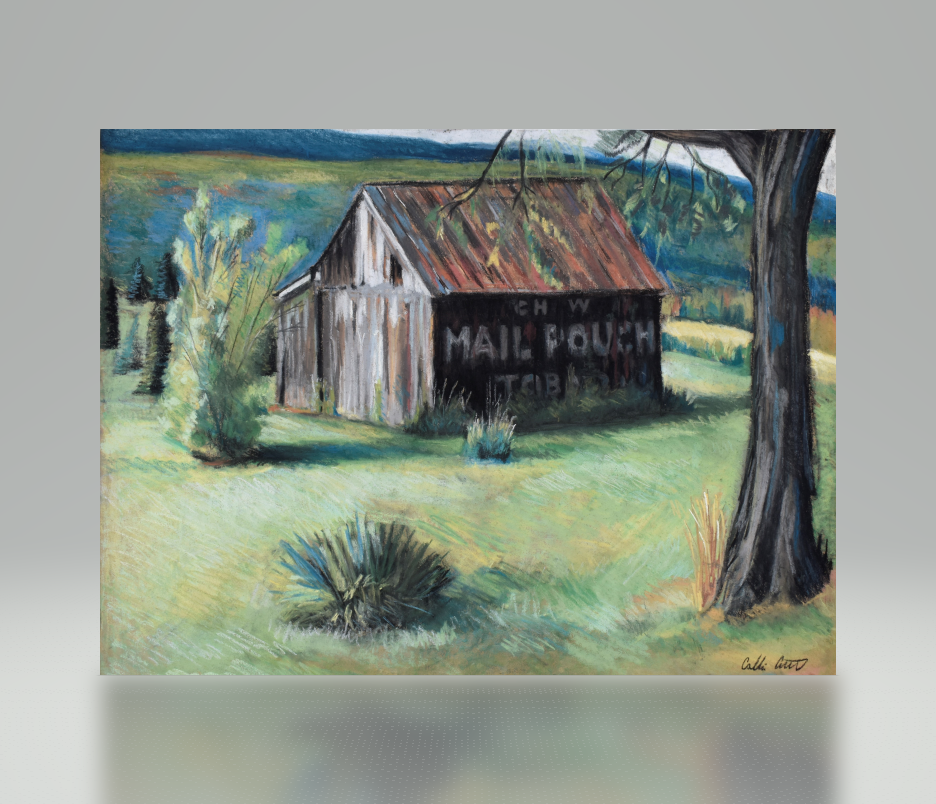In the center of the painting, a brown wooden barn with a slanted roof is prominently featured, bearing the white lettering "CHW" and large letters spelling "MAIL POUCH" underneath. The painting is surrounded by a thick gray border, creating a frame for the lush, vibrant scene. To the left of the barn, there is a big green bush, while towards the right side, a tree stands with a sparse canopy of green leaves. In the background, a verdant hillside composed of green and blue hues sets a serene pastoral scene, accentuated by five trees scattered across the landscape. The ground is covered in lush green grass, and a small bush is visible near the bottom of the painting. The artist's signature, "COCKGOOD," is inscribed in script in the bottom right corner of the border.